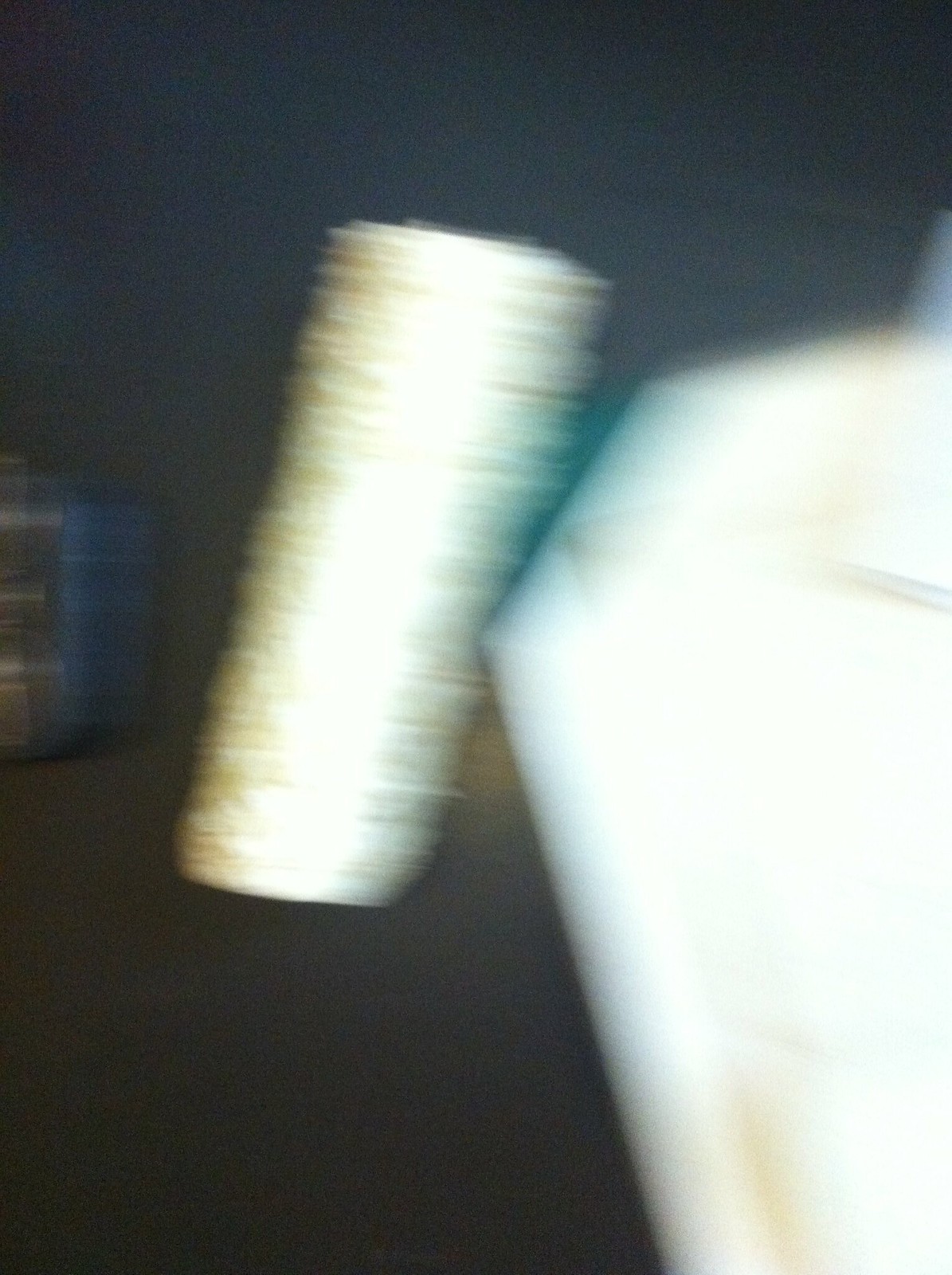The image appears to be significantly blurry and grainy, making it challenging to discern specific details with complete certainty. The dominant feature is a pair of light objects against a dark background, likely taken at night. On the left, there's a fuzzy, rectangular light that might resemble a painting brush or a faint fluorescent light. There's also a blue, cuboid object on the left that could be a vending machine, though it is indistinct. The right side of the image features a large, angular, white shape that extends from the bottom right towards the center, possibly indicating a metal canister or cylinder adhered to a white appliance. This central object shows some striated gray and brown areas. The overall scene includes dark lines, reflections on an orange-brown ground, and a vague suggestion of a dental chair perspective, adding to the complexity and ambiguity of interpreting the image.